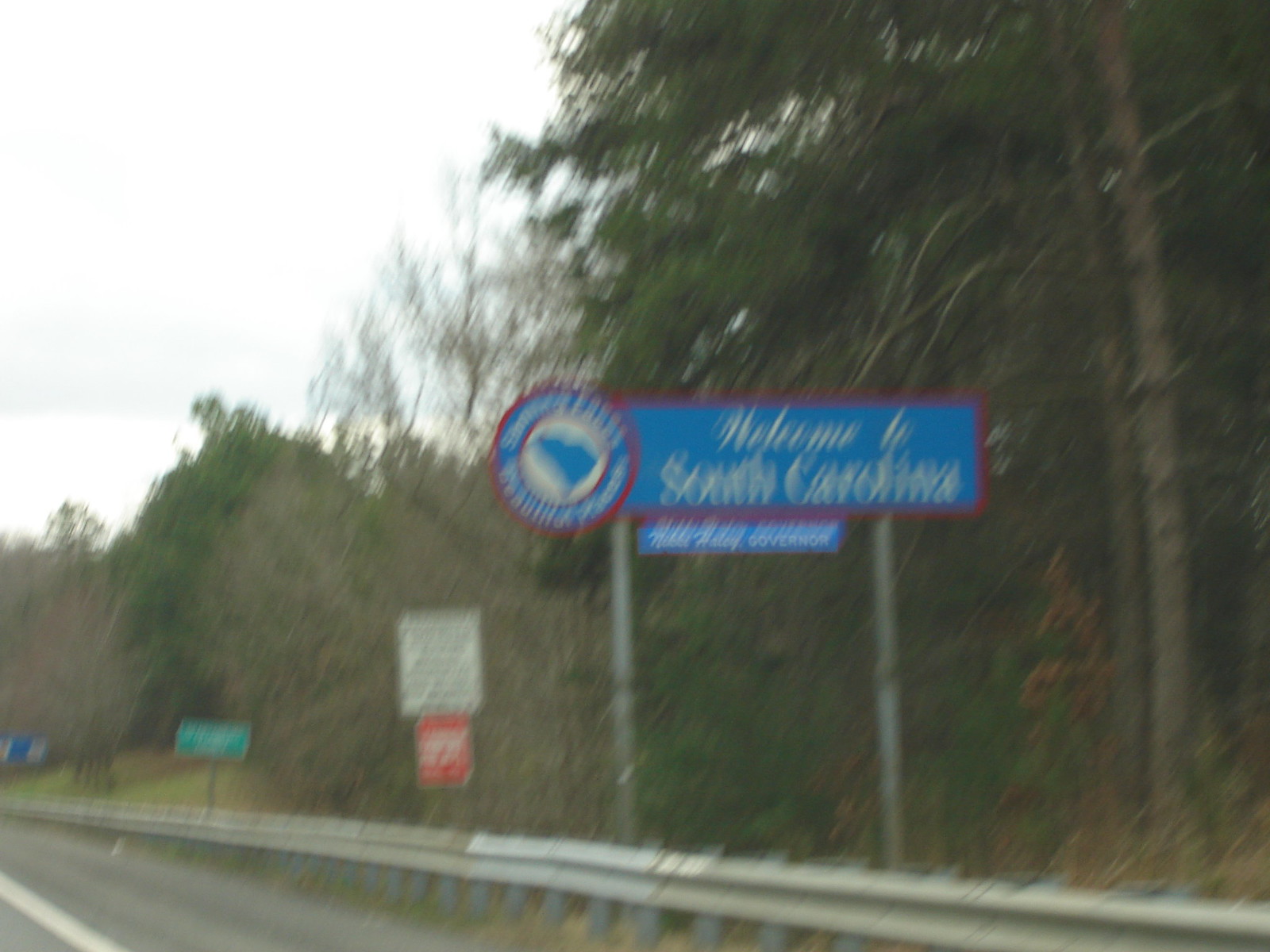The photo, taken during the daytime and slightly blurry as if captured from a moving car, depicts a highway scene with multiple signs and roadside elements. Dominating the image is a large rectangular blue sign with a maroon or red outline, supported by two posts, reading "Welcome to South Carolina" in white lettering, accompanied by a blue silhouette of the state within an inner white circle. Adjacent to the blue sign, on the right side, you can see a white rectangular sign with black text and a smaller red rectangular sign with white text beneath it. To the left of these signs, there is a typical green highway sign, likely indicating a creek or mile marker. A silvery-gray guardrail, supported by wooden or steel posts, runs along the side of the road from the bottom right of the image, accompanied by a visible white sideline marking the shoulder of the highway. The background features a slightly uphill, heavily wooded area with a mix of green and brown hues.